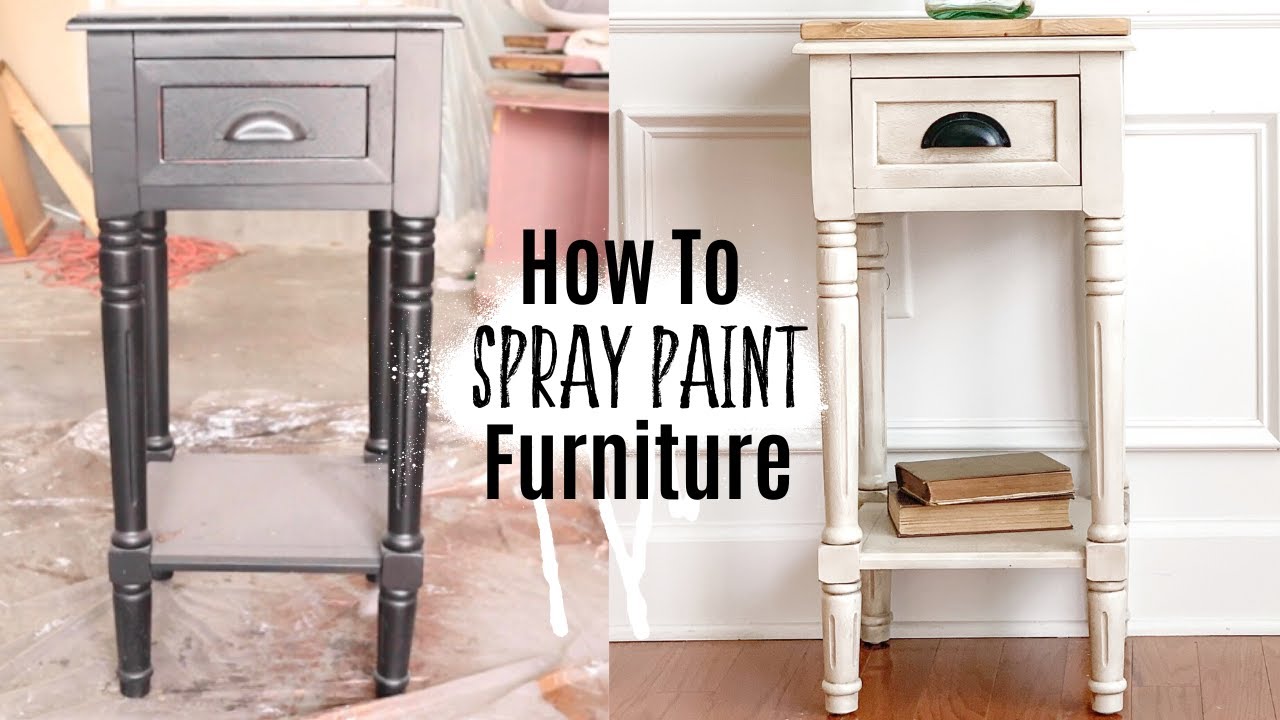The image is a detailed graphic titled "How to Spray Paint Furniture," featuring a side-by-side transformation of a tall, narrow side table or nightstand. On the left, the "before" photo shows the nightstand with a gray drawer, a silver handle, four darker gray legs, and an additional gray board near the bottom. The piece is situated on protective paper, likely for the painting process. The right "after" photo presents the nightstand painted in a rustic, creamy white, with a now black, solid arch handle that allows for easy gripping. The bottom shelf displays two old books, and the staging includes a wood piece on top, all set against a white wall with a brown floor, indicating the transformation's completion inside a home.